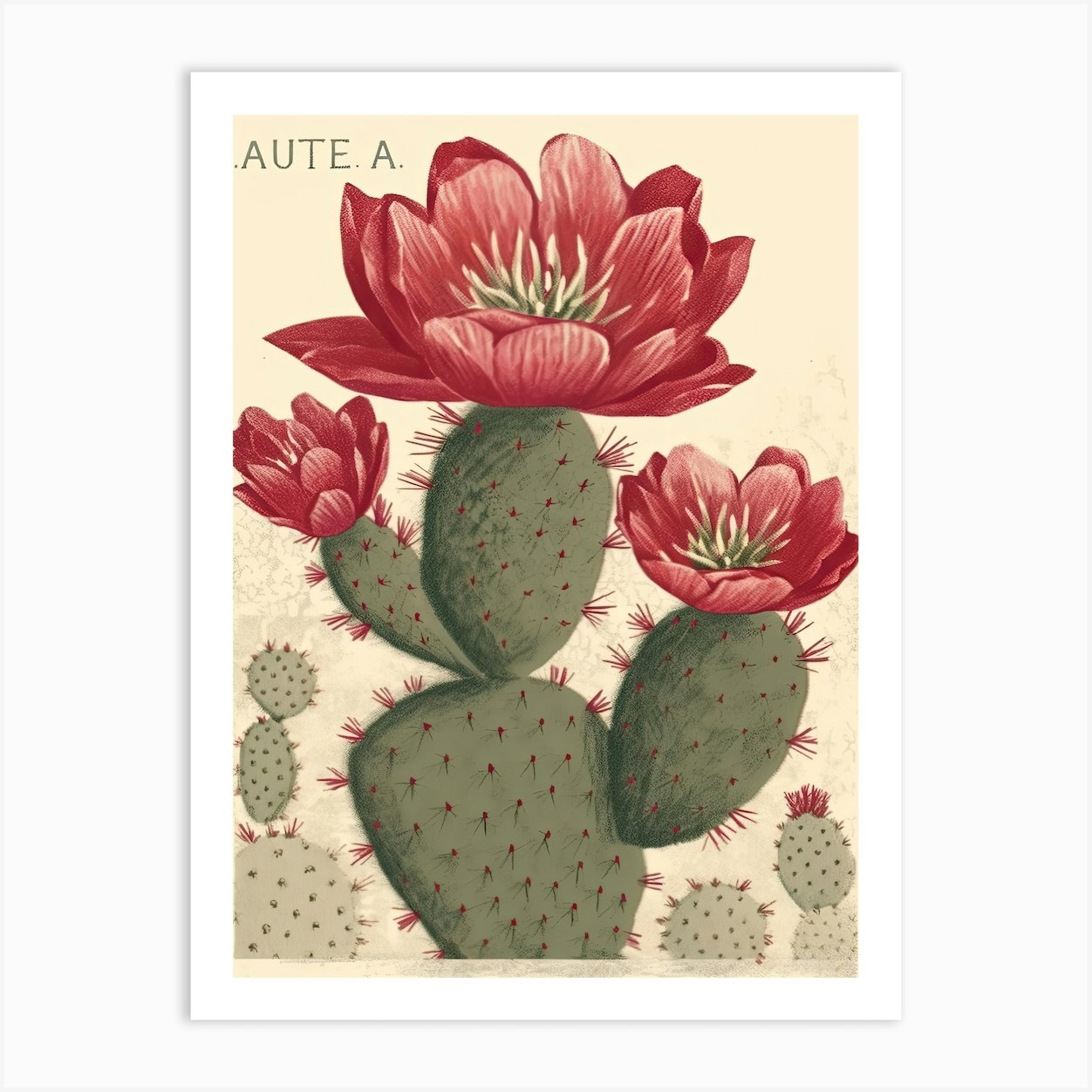This is a detailed illustration, possibly a vintage greeting card or a botanical print, depicting a cactus in bloom against a soft yellow or beige background. The illustration features a large central cactus characterized by stacked, roundish pads covered in maroon to blood-red needle-like spines. Three red flowers, varying in bloom stages—one barely open, one partially open, and one fully open—adorn the tops of these pads, each flower displaying layered petals with a green to light yellow center.

The image also includes several smaller cacti of the same species in the background and lower sections, each adorned with similar red spines and flowering buds. The entire scene is framed with a white border, and the top of the piece is labeled "AUTE.A" in uppercase letters, possibly indicating the name of the cactus. The styling and composition suggest the illustration could have been a plate in an old book of botanical illustrations or a print used for greeting cards or postcards.